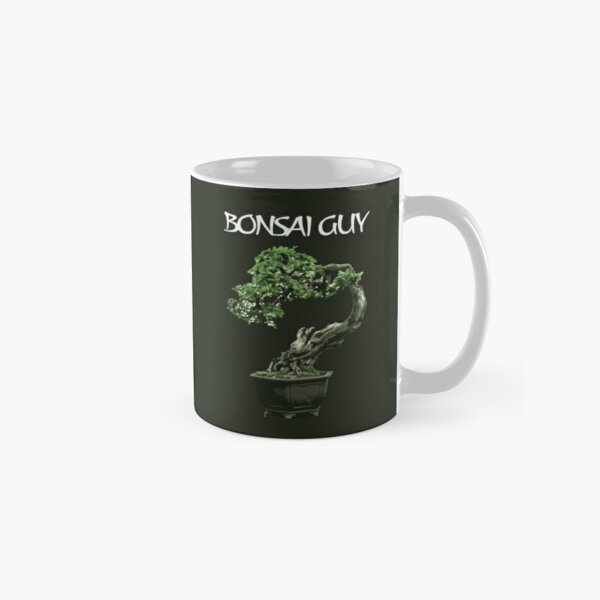The image depicts a dark green coffee mug with a white interior and a white handle, positioned against a plain off-white background. The mug features a centered illustration of a bonsai tree growing out of a dark-colored pot. The bonsai tree has a thick trunk that curves to the left and is adorned with green leaves. Above the image, in white, Asian-style font, the text "Bonsai Guy" is prominently displayed. The label does not extend around the entire mug, with some white visible near the handle.